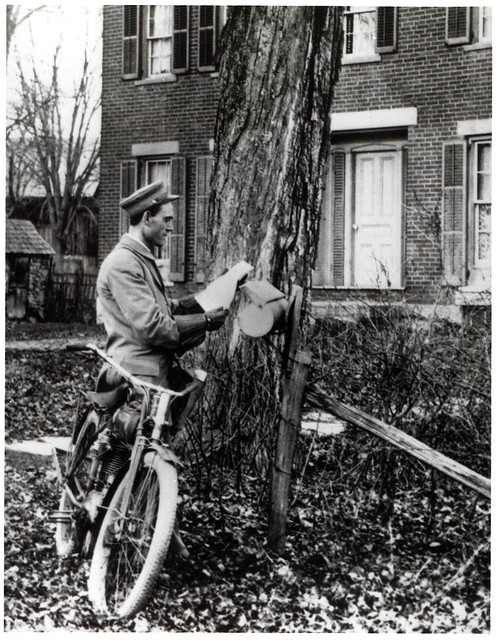In this black and white photograph, a man in an old-fashioned, possibly postal or military, uniform stands with a bicycle leaning against him as he reads an unfolded letter. He wears a hat, a heavy coat, and large gloves, suitable for a chilly day. The ground is littered with fallen leaves, suggesting late fall or winter. In the background, there is a tall, leafless tree, and beside it stands a tall metal container on a post, likely a mailbox. The scene unfolds in front of a two-story brick building with several windows adorned with slatted shutters and a white front door, accessed via steps. To the left, another tree and more buildings are visible, enhancing the scene's nostalgic feel.